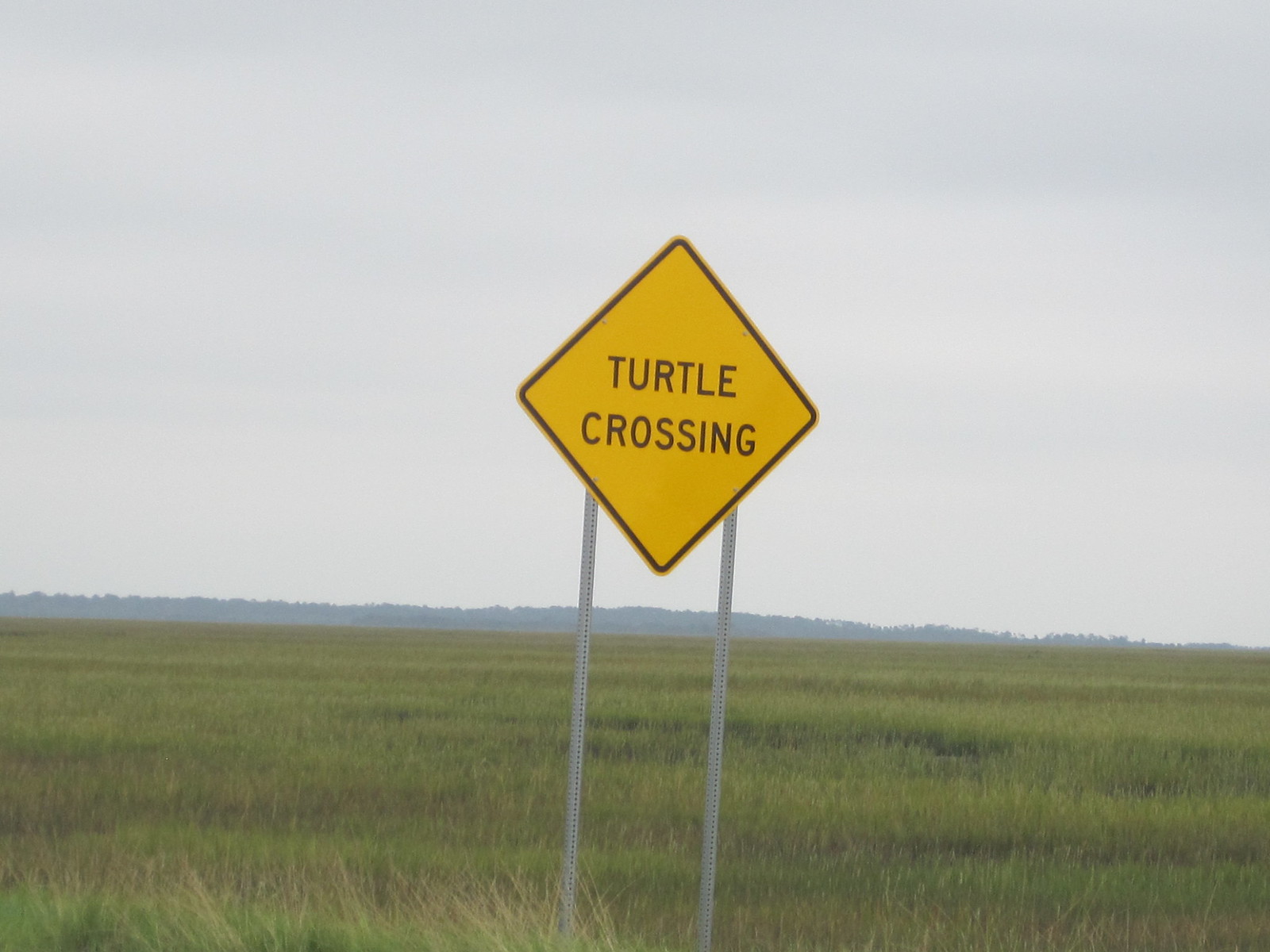A stunning photograph of exceptional quality prominently features a yellow and black "Turtle Crossing" sign mounted on a silver metal post, positioned almost dead center in the image. The sign has a golden yellow background with black lettering and is bordered by a thin black line. Surrounding the sign is a patch of thick, lush grass displaying various shades of green, interspersed with patches of brown. The background reveals a heavy tree line under a gray sky, adding depth and context to the scene. The image is remarkably clear and detailed, capturing the essence of a serene, natural environment.